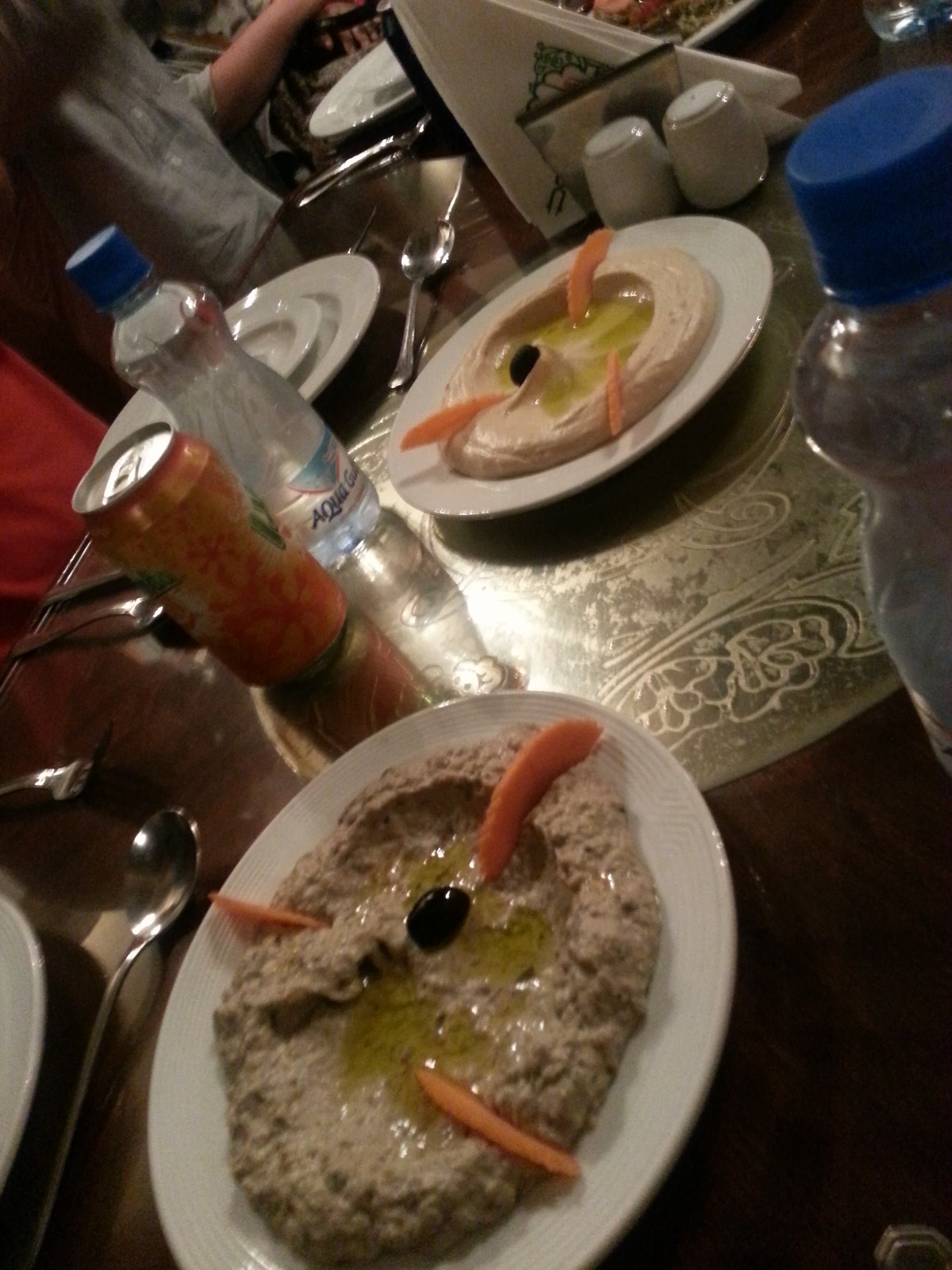The image depicts a slightly angled restaurant table setting adorned with various items. Central to the foreground are two white plates, each featuring a meticulously arranged serving of what appears to be hummus. The hummus on each plate is fluffy and beige-brown, garnished with a black olive placed at the center, and has thin slices of fruit or vegetable, possibly carrots, arranged around. One serving is slightly lighter in color compared to the other. Behind these plates, we see a bottle of water and an orange soda can. Additional details include inverted cups in the distance, typical restaurant plates, utensils, and a napkin holder. Salt and pepper shakers are also visible. There's an individual seated at the table in the background, with only an arm visible, likely signifying other's presence or dining company. The overall image is slightly out of focus, contributing to its casual, candid nature.